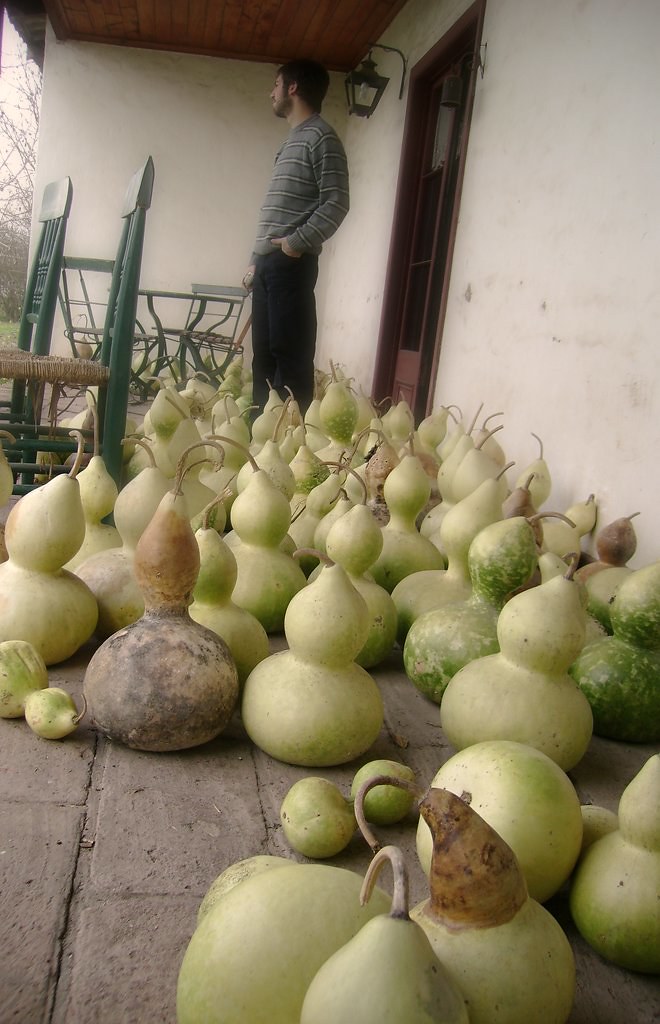The photograph captures a rustic front porch with a gray brick floor, adorned with an abundance of uniquely shaped gourds. These gourds, resembling two-tiered snowmen, display a palette ranging from off-white to lime green, with some featuring darker green hues. Scattered throughout the scene, a few brown gourds add to the autumnal atmosphere. Occupying the right side of the porch, a man with dark brown hair and a beard stands, dressed in black pants and a gray shirt with black and white stripes. His left hand rests in his pocket as he gazes to the left. Behind him, a wooden door fitted with glass panes is partially visible. Mounted to the wall beside the door is a black lamp, casting a quaint light over the setting. To the left side of the porch, a small round metal table is paired with two green ladder-back chairs featuring brown wicker seats, adding to the cozy charm of the scene.